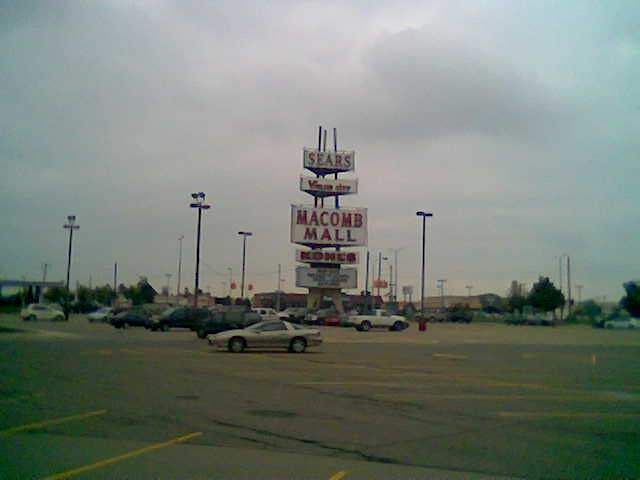This image depicts a sparsely occupied parking lot at a mall. The asphalt surface of the lot appears aged and weathered, bearing visible cracks and stains from previous vehicle drips. The yellow lines marking the individual parking spaces are prominent in the foreground. 

Among the parked vehicles, there's a gray sports car, followed by various sport utility vehicles in white, black, and other colors. A white pickup truck is also present. 

In the background, a large, multi-post sign towers over the scene. At the top, the sign prominently displays “Sears” in a bold white banner with red lettering. Below it, another unreadable sign is positioned. The largest section of the sign reads “McComb Mall,” with “Kohl’s” listed beneath it, indicating the mall's prominent retailers.